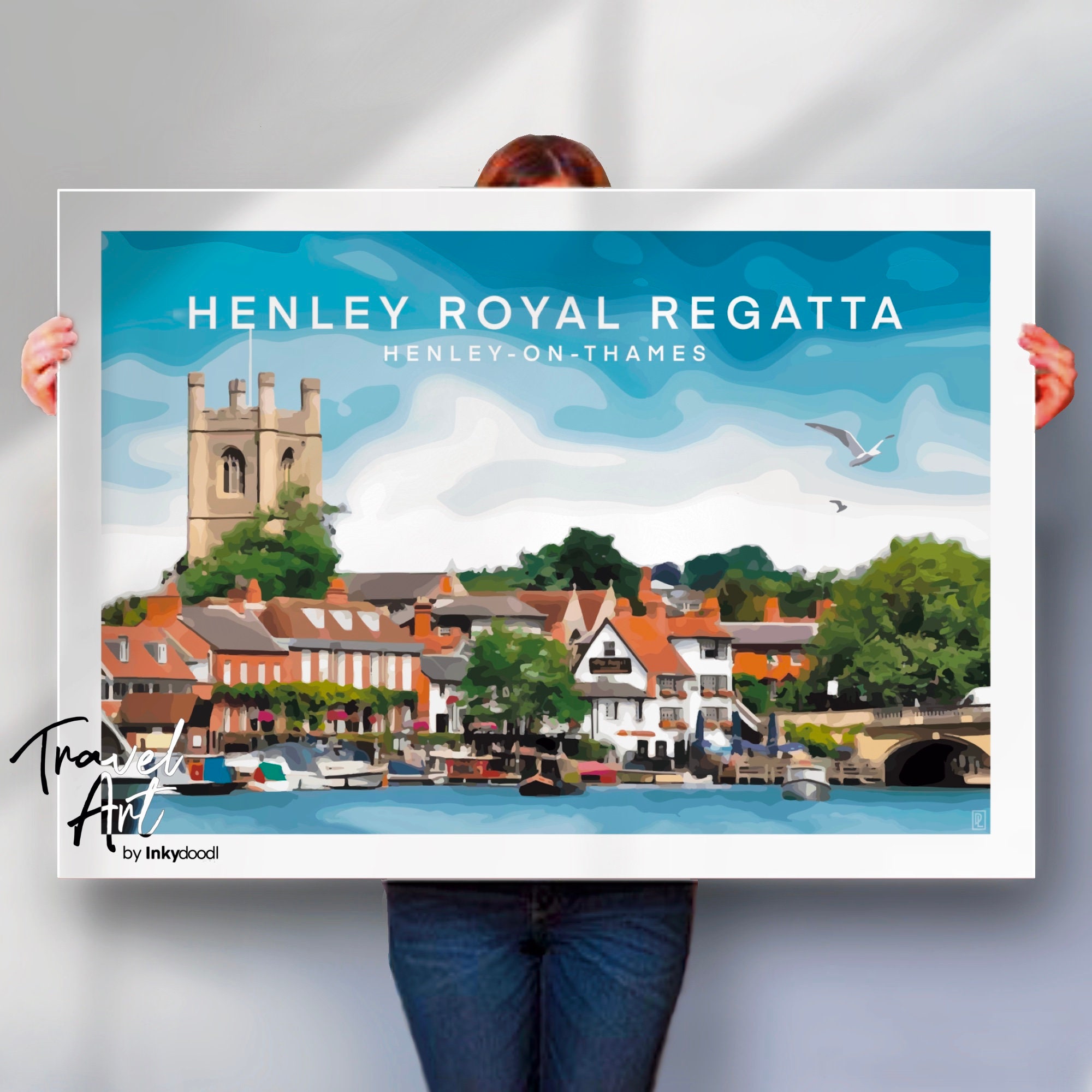In this image, a woman with red hair, parted in the middle, is holding up a painting. The painting, labeled "Henley Royal Regatta" at the top, also features the words "Henley on the Thames" below it. The artwork depicts an old English village with boats and canals, including a prominent bridge with a tunnel and a big tower topped with turrets. The town features distinctive orange brick buildings and a white structure, set alongside a row of houses by a bay. Scattered boats can be seen throughout the scene. The bottom left corner of the painting is signed "Travel Art by Inky Doodle." The woman, whose face is not visible in the image, is holding the painting with her hands on either side, and you can see her legs from the crotch down, dressed in blue jeans.